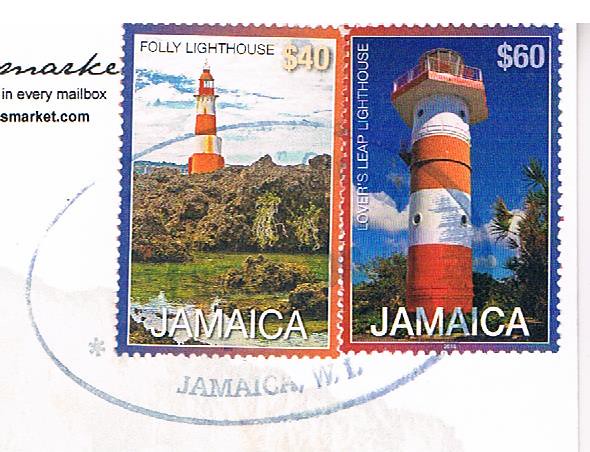The image showcases the top right corner of a postcard, prominently featuring two vividly colored postage stamps side by side, each depicting iconic lighthouses. The postcard also has a caption photoshopped onto it, reading, "Mark, in every mailbox market.com," suggesting it's an advertisement for purchasing stamps. 

The left stamp, valued at $40, depicts the Folly Lighthouse in Jamaica. It features a striking red and white lighthouse perched on a rocky, vegetated edifice by the seaside, with a glimpse of green water at the base of the rocks. The sky in the background showcases a few clouds, adding to the picturesque scenery.

The right stamp, priced at $60, presents the Lover's Leap Lighthouse, also in Jamaica. This lighthouse is similarly styled in red and white, viewed from a low angle, accentuating its grandeur. Behind the lighthouse, some trees and a bright blue sky with sparse clouds can be seen.

Both stamps share a colorful border and are marked with "Jamaica" in white lettering at the bottom. A rubber stamp impression on the postcard gives the appearance that it has been mailed, emphasizing the authenticity of the advertisement.